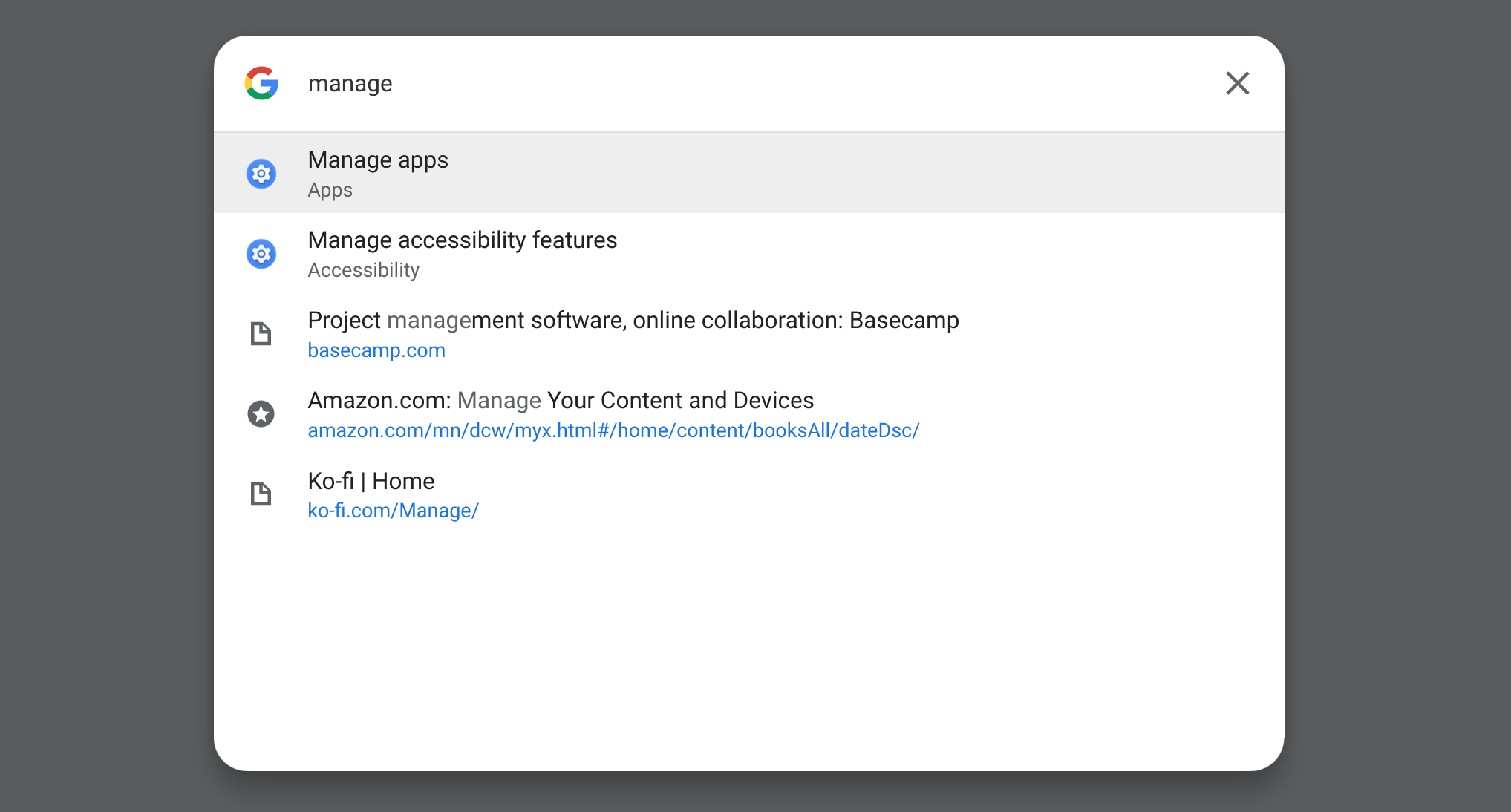A Google search result is displayed in the middle of a smartphone screen, where the term "manage" has been queried. The results include both phone settings and various websites. On the phone, search results highlight "Manage app settings" and "Manage accessibility features". Web-based results list well-known sites: Basecamp with "Project management software", Amazon with "Manage your content and devices", and Ko-fi with "ko-fi.com/manage" in the URL. The screen background is a mix of white and gray, indicating it might be on a launcher or relevant search page. Various links and settings emphasize the utility of different management features on both the device and the web.